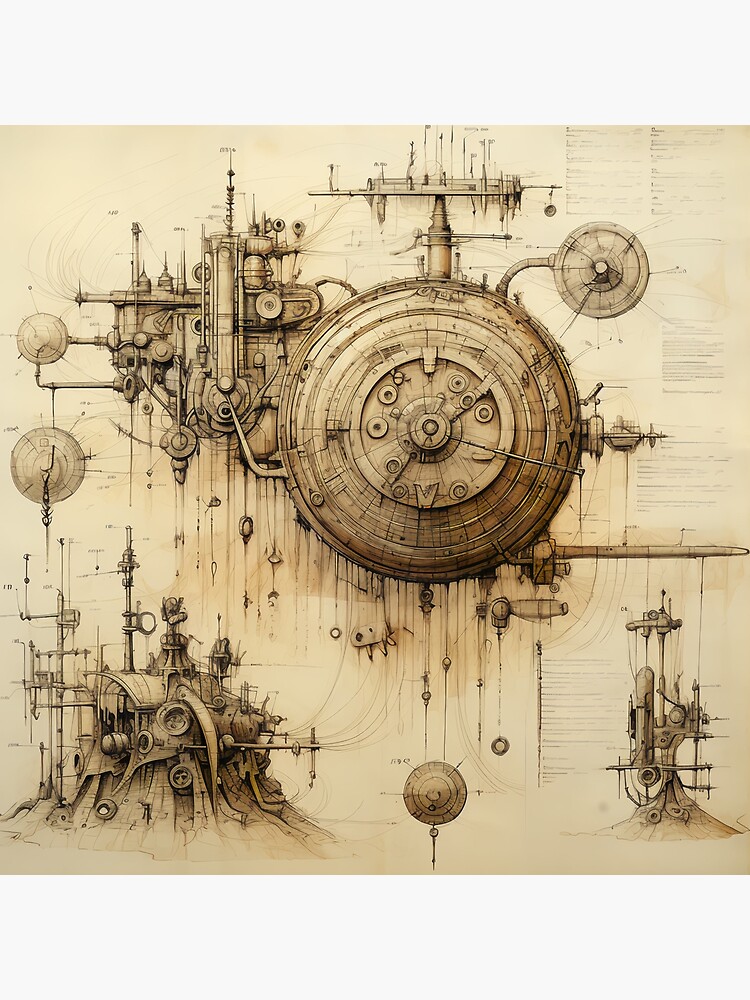A detailed steampunk illustration on antique-style paper. The brownish-tan paper has hints of orange, giving it an aged appearance. The intricate drawing features a large, circular device resembling complex machinery that appears both futuristic and antique, contributing to its steampunk aesthetic. This central circular object is adorned with numerous platforms, lines, and gadgets, and is suspended by straight lines attached to circular pendants, suggesting that the device might be flying in the sky. The image is filled with tiny, unintelligible prints and lines connecting different parts, resembling a technical diagram.

In the lower right-hand corner, an oblong device emerges from the ground, clearly man-made with numerous antennas and straight platforms extending from its sides. In the lower left-hand corner, another building ascends from the ground, combining a futuristic outer-space look with an old, antique feel. This structure is covered in antennas, spikes, and gear-like circles that could be windows, creating a sharply detailed and mechanical appearance. Thin, delicate lines resembling cords or electrical wires rise from the buildings and connect to the central mechanical ship, enhancing the interconnected intricacy of the entire illustration.